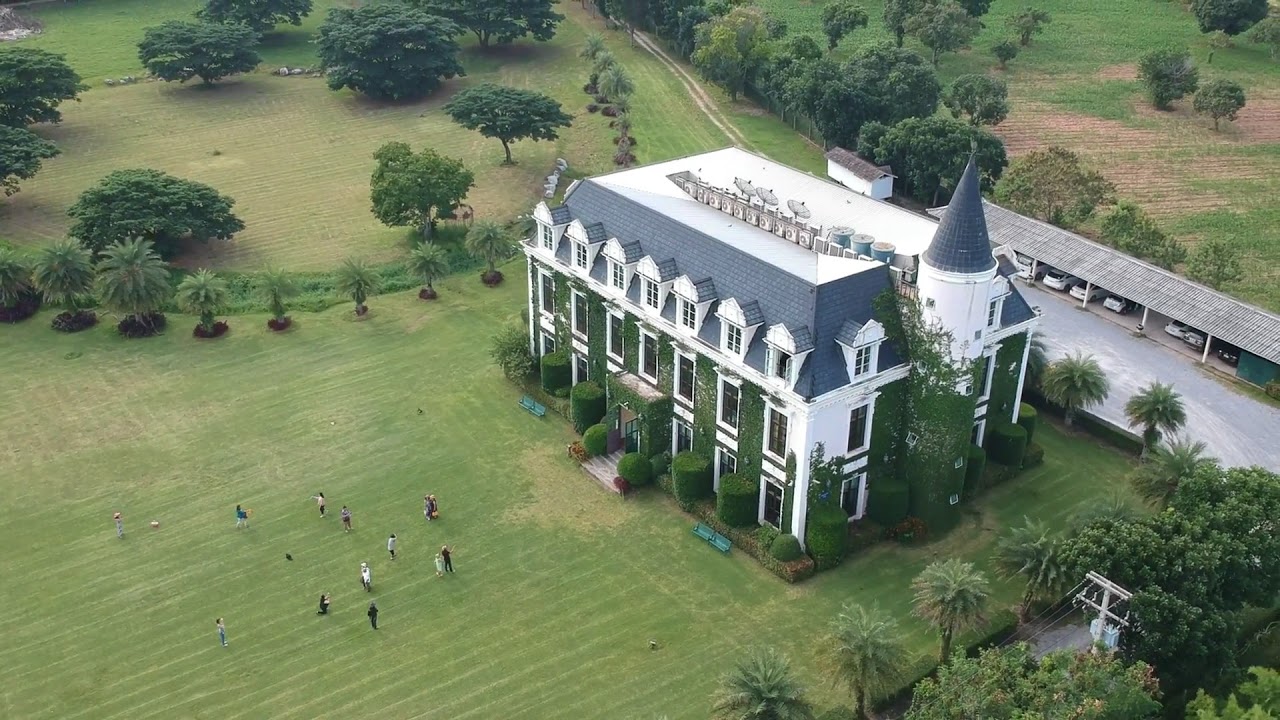This aerial shot captures a picturesque three-story mansion with a distinctive navy blue and white exterior. The building boasts a unique conical tower on one side and an array of satellite dishes atop its roof. The surrounding landscape features a meticulously manicured lawn mowed by a lawnmower, punctuated by professionally trimmed shrubs and palm trees. There is a notable presence of greenery, including scattered trees throughout the property. In front of the mansion, approximately ten to twelve individuals are gathered on the field, which also houses several benches for seating. The expansive property extends over a few acres, encompassing an outdoor garage with an awning sheltering multiple cars, predominately white, and one dark-colored vehicle. Additionally, a dirt path meanders through the landscape, leading to a shed visible in the distance.